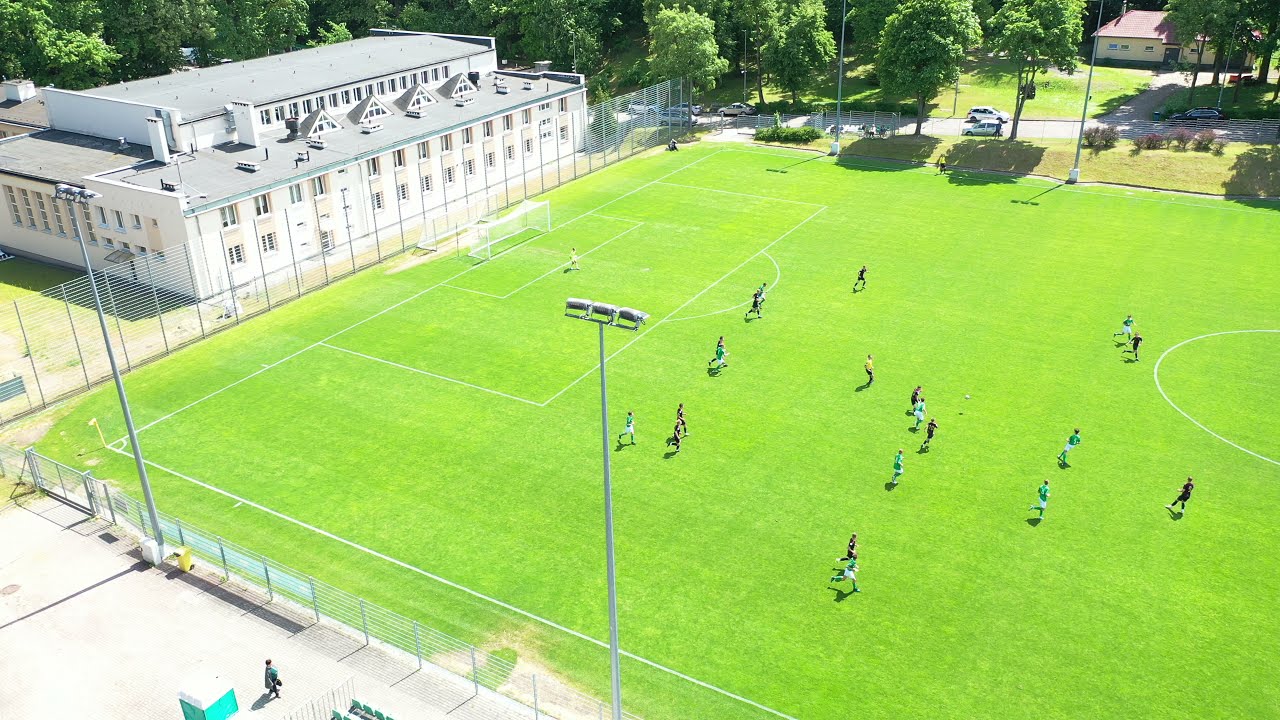This aerial photograph captures a lively soccer match in progress on a sprawling, bright green field under a sunny sky. The players, distinguishable by their light and dark-colored uniforms, are dynamically scattered across the field, with the ball visibly in the air. White lines and circles mark the well-maintained grassy surface in accordance with soccer regulations. Surrounding the field is a tall cyclone fence, and beyond it, trees line the area, adding a touch of nature to the scene. A prominent white, three-story building, likely a school or gymnasium, stands at the upper left corner of the image. Adjacent to this building, a gravel road and parking lot are partially visible. To the side of the field, a street with cars parked and driving flanks the area, indicating a neighborhood setting. Towering stadium lights loom over the scene, ready to illuminate evening games.